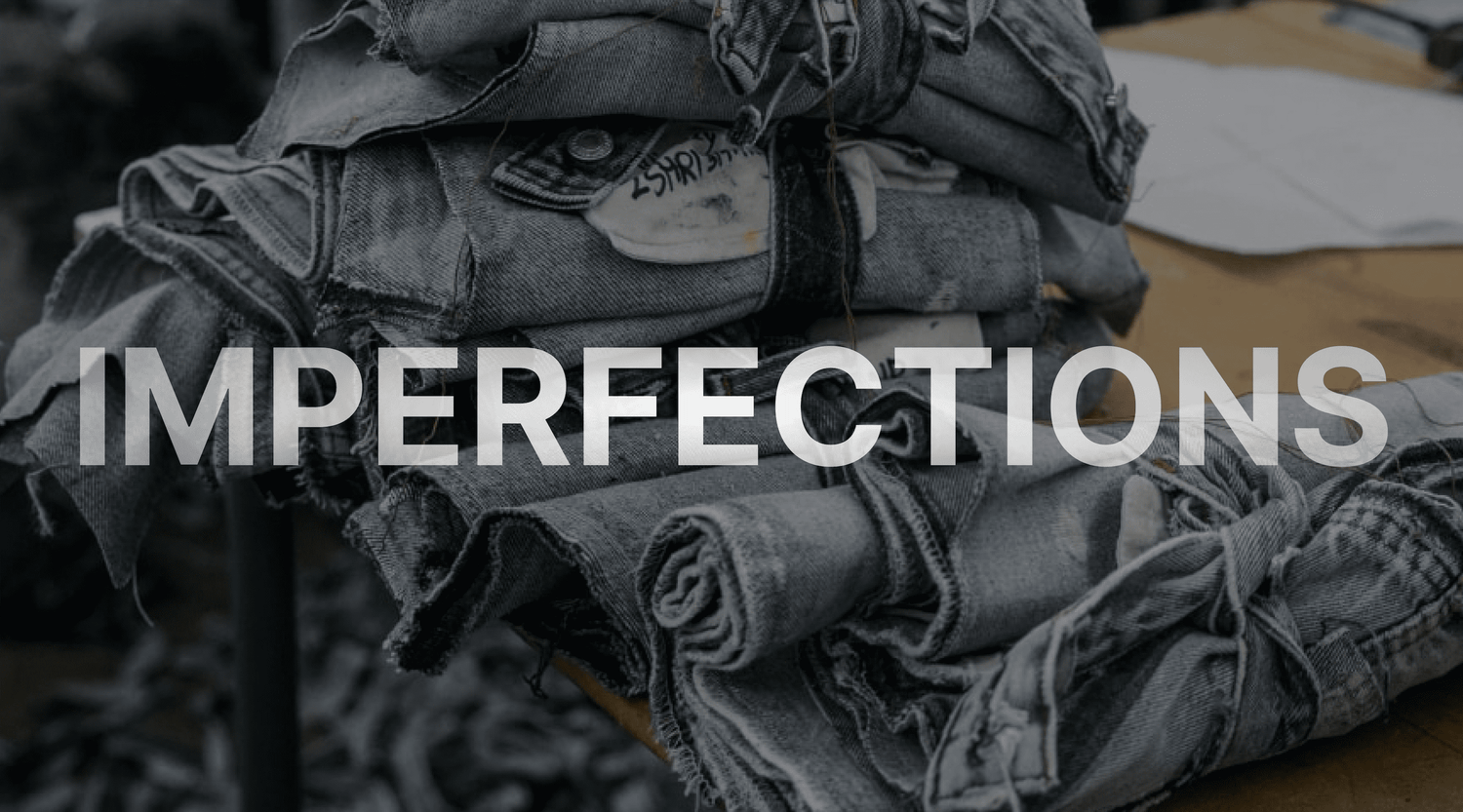The image is a horizontally rectangular indoor photograph with a desaturated, almost black-and-white color palette. At the center, a light wooden table is piled with various heavily deconstructed, rolled, and tied denim pieces — primarily blue jeans, but possibly also denim jackets or shirts. These denim items are arranged from the middle top, cascading diagonally to the right side of the image. Above this heap of denim, stretched across the middle in bold, white lettering, is the word "Imperfections." Along the right edge of the table, there are some papers visible, while to the left, a black table leg descends out of the frame. The background is blurry, dominated by dark colors, possibly carpet or a rug in the lower left, and additional piles of denim scraps scattered on the floor.